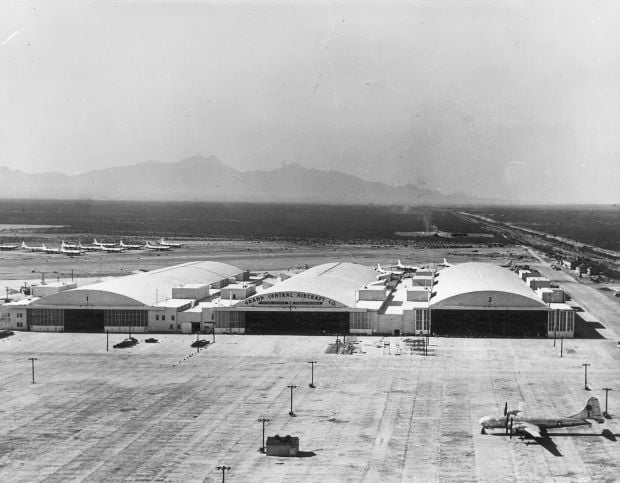This black-and-white aerial photograph, likely taken decades ago, depicts an old airport airfield with three long, white airplane hangars prominently displayed in the center. The middle hangar bears the name "Grand Central Aircraft Company." The expansive parking lot in front of the buildings is mostly empty, save for a few cars towards the upper left and a small building centrally located within it. Rows of streetlights align the parking area. On the right of the lot, an old, white airplane is parked, and further back, towards the left, there is a fleet of aircraft, all seemingly idle. The backdrop features a grassy area leading up to mountain ranges, under a cloud and gray sky, enhancing the historic and grainy feel of the photograph.